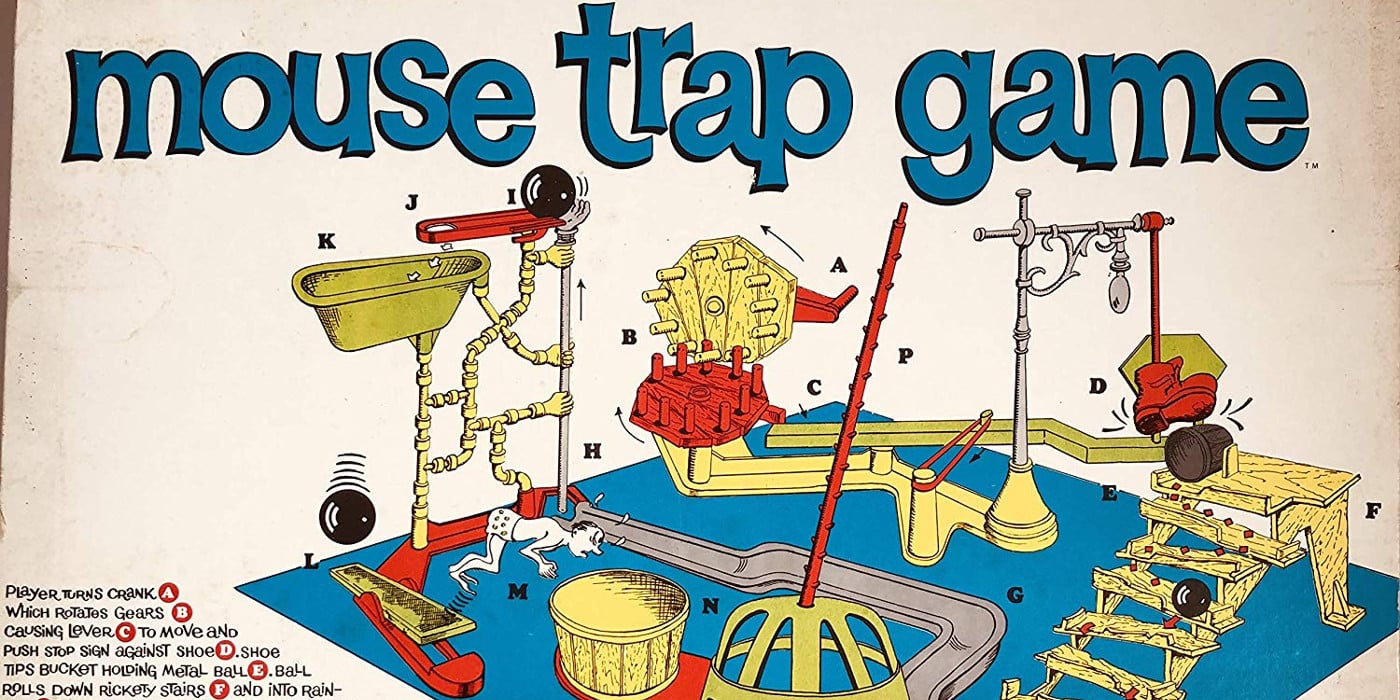The image is a detailed photograph of the box cover for the board game "Mousetrap Game." At the top of the box, large blue letters spell out the game's name. Beneath this title is an intricate diagram illustrating how the game is set up, with each piece labeled and described. Central to the game's mechanics is a Rube Goldberg machine: the instructions start with a player turning a crank (labeled A), which rotates connected gears (B). This in turn moves a lever (C) to push a stop sign against a shoe (D). The shoe tips a bucket (E) holding a metal ball, which then rolls down a series of rickety stairs (F). The rest of the sequence involves the ball eventually triggering additional parts of the machine. This engaging and whimsical process is designed to trap the mouse, with each component meticulously interconnected to achieve the final goal. The box cover displays all components with corresponding lowercase letters, making it clear and visually descriptive for players.